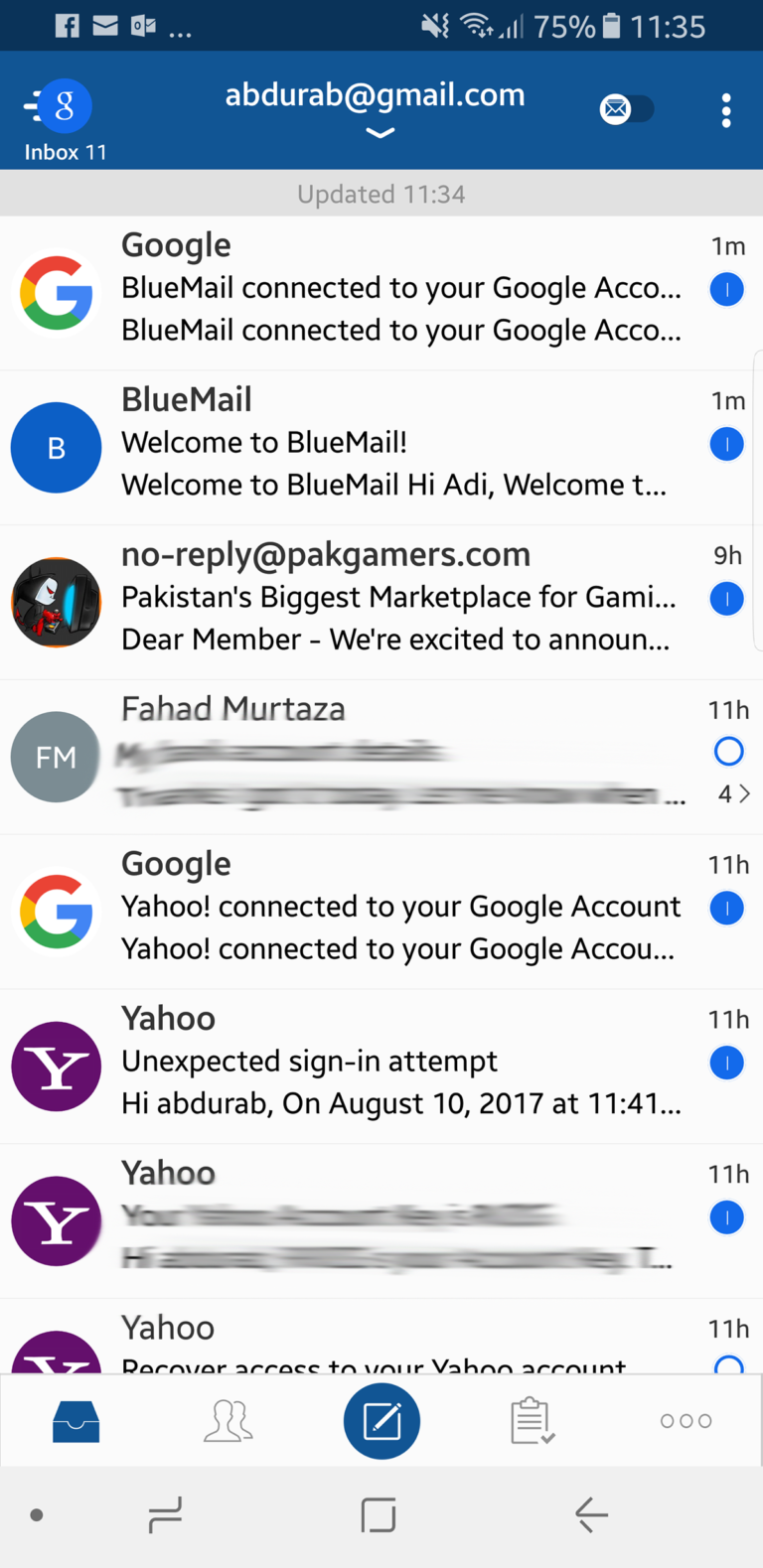The image depicts a mobile phone screen displaying the Gmail inbox of the user abderab@gmail.com. The present time is 11:35 AM, and the phone is at 75% battery. At the top of the screen, there are icons for Facebook and email notifications. 

The Gmail app interface is characterized by a blue header that indicates the inbox was last updated at 11:34 AM. The inbox contains 11 messages.

1. The first email is a Google notice with the G logo, informing about Blue Mail's connection to the user's Google account.
2. The second email is from Blue Mail, offering a welcome message to the service addressed to "Hi Addy," though the content snippet is partially cut off.
3. The third email is from no-reply@packgamers.com, which appears to be from Pakistan's largest gaming marketplace, but the content is truncated.
4. The fourth email, from Fahad Murtaza, is blurred, preventing any content from being read.
5. The fifth email is another notice from Google about Yahoo being connected to the user's Google account.
6. The sixth email is from Yahoo, stating there was an unexpected sign-in attempt on August 10th, 2017.
7. The seventh email, also from Yahoo, is blurred and the content is not visible.
8. The last visible email subject is from Yahoo, providing information on how to recover access to the user's Yahoo account, but it is cut off.

At the bottom of the screen, there are standard email icons including options to compose a new email, potentially manage contacts, and store older emails. Additionally, there are the standard phone navigation buttons: a home button, a back button, and a task manager button.